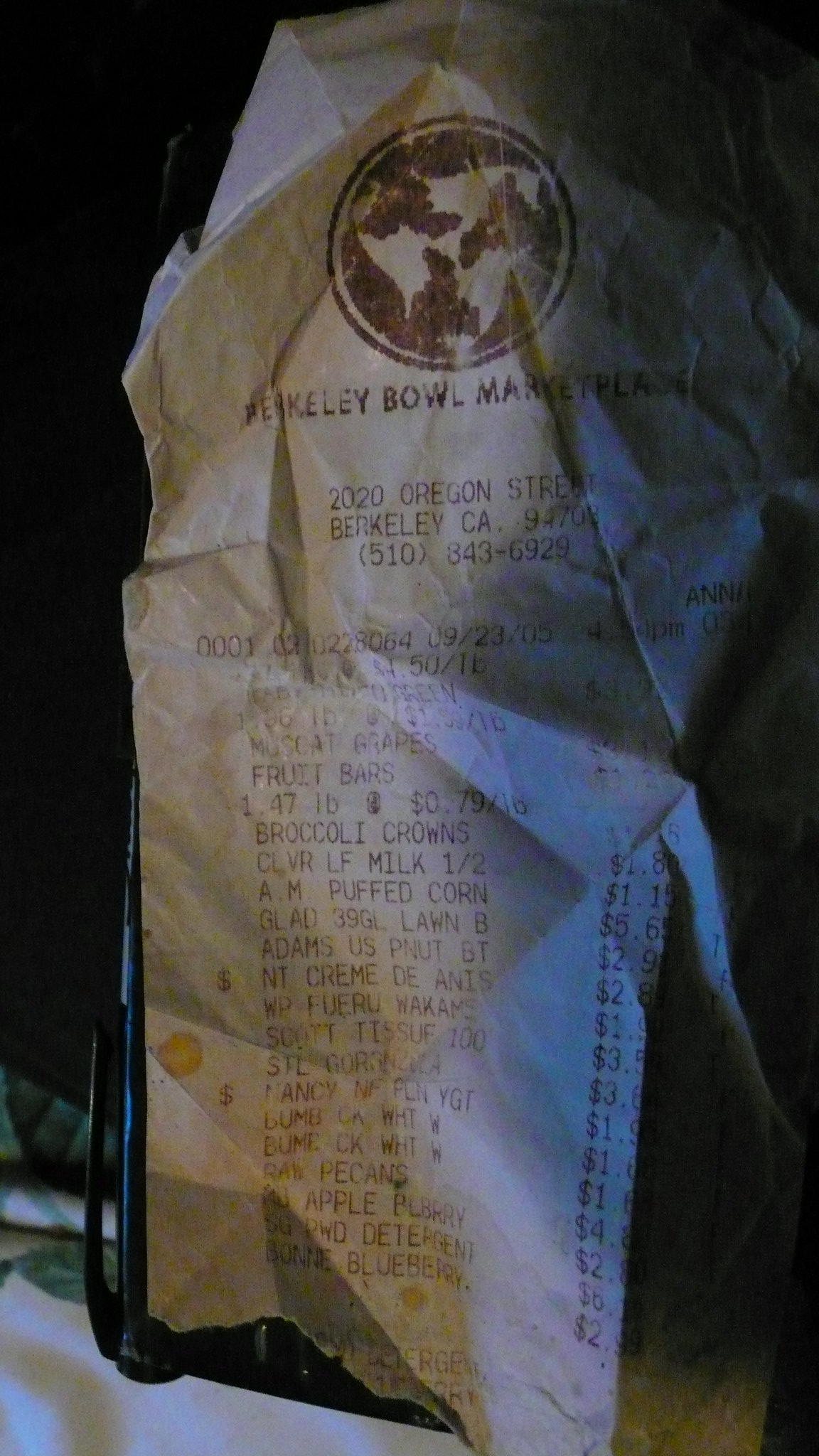In this vertical, rectangular image, we are presented with a detailed photograph of a black tray, reminiscent of those used in restaurants to present receipts or bills. The tray prominently features a stark white receipt, which appears aged or water-damaged since some of the printed text is faded and blurred. At the top of the receipt, there's an image of the Earth, with continents depicted in white against a black background. Directly below this, the text reads "Berkeley Bowl Market," followed by the address "220 Oregon Street, Berkeley, California" and the contact number "510-843-6929." 

Further down, various line items are discernible, listing: 
- Muscat grapes
- Fruit bars
- Broccoli crowns
- Cloverleaf milk, half gallon
- Glad lawn bags, 39 gallon
- Adams peanut butter
- Nancy's plain yogurt
- Apples
- Blueberries
- PWD powder detergent

However, the total amount on the receipt is illegible as only partial numbers are visible, with the first digit missing.